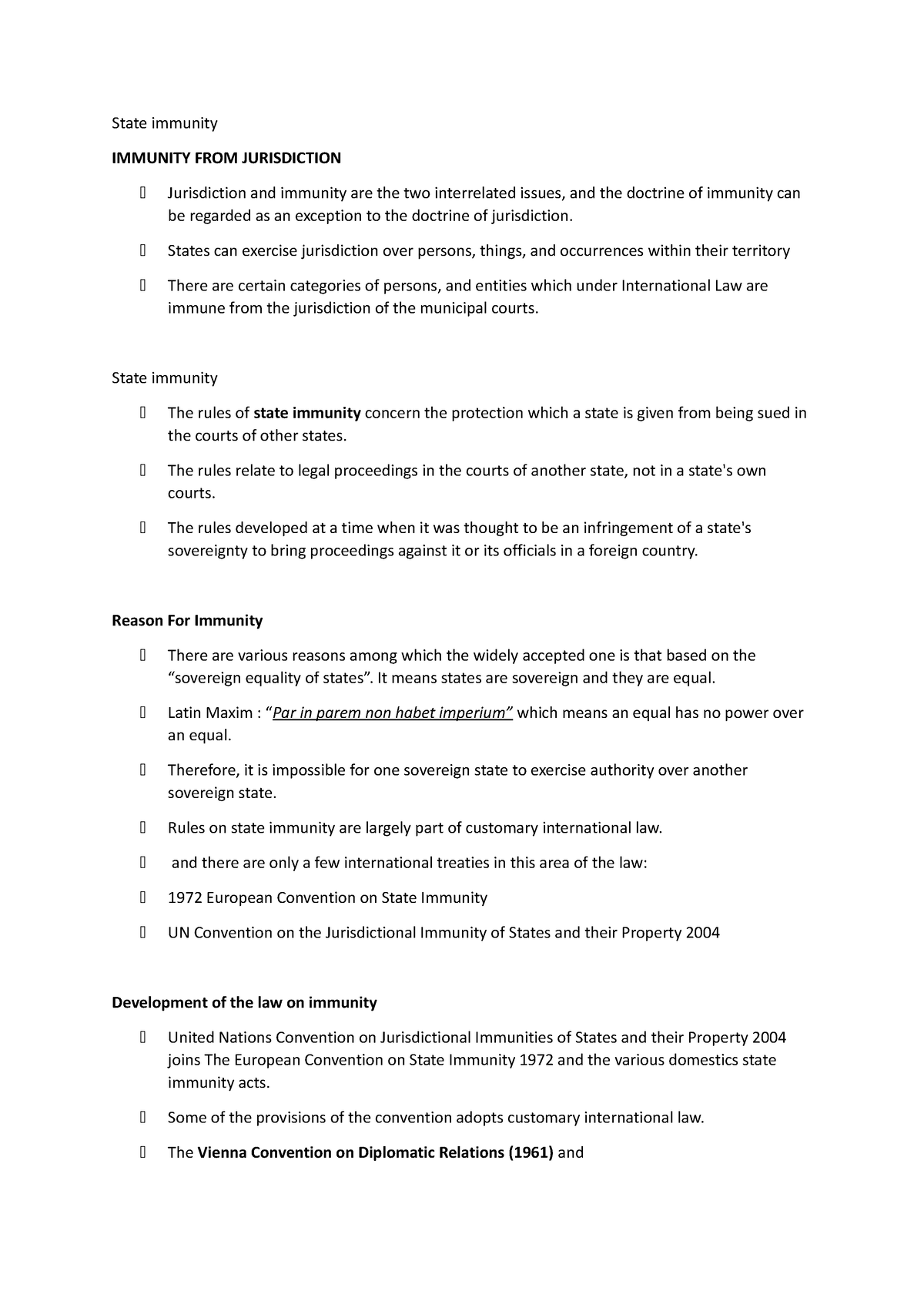The image displays a typed document, likely from courtroom notes or a legal reference, set against a white background with black font. The document is structured with headings, bullet points, and sections highlighted in bold for emphasis.

**1. Heading: State Immunity**  
The document begins with a main heading, "State Immunity," which introduces the topic.

**2. Subheading: Immunity from Jurisdiction (Bold Font)**  
This subheading is emphasized in bold.

**3. Bullet Points under Immunity from Jurisdiction:**  
   - **First Bullet Point:** "Jurisdiction and immunity are two interrelated issues. The doctrine of immunity can be regarded as an exception to the doctrine of jurisdiction."
   - **Second Bullet Point:** "States can exercise jurisdiction over persons, things, and occurrences within their territory."
   - **Third Bullet Point:** "There are certain categories of persons and entities which, under international law, are immune to jurisdiction in municipal courts."

**4. Subheading: State Immunity (Bold Font)**  
Another bold subheading follows, reiterating "State Immunity".

**5. Bullet Points under State Immunity:**  
   - **First Bullet Point:** "The rules of state immunity (with 'state immunity' in bold font) concern the protection given to a state from being sued in the courts of other states."
   - **Second Bullet Point:** "The rules relate to legal proceedings in the courts of another state, not in a state's own court."

**6. Subheading: Reasons for Immunity (Bold Font)**  
Highlighted in bold, this subheading introduces a section listing reasons for immunity.

**7. Bullet Points under Reasons for Immunity:**  
   - There are seven bullet points, though the exact text of these points is not detailed in the brief.

**8. Subheading: Development of Law on Immunity (Bold Font)**  
This bold subheading suggests another section, which discusses the development of law concerning immunity.

**9. Bullet Points under Development of Law on Immunity:**  
   - There are three bullet points, with topics such as the United Nations Convention provisions among others.

The document appears comprehensive, covering various aspects of state immunity, including its relationship with jurisdiction, specific rules, reasons for immunity, and its development through international legal frameworks.